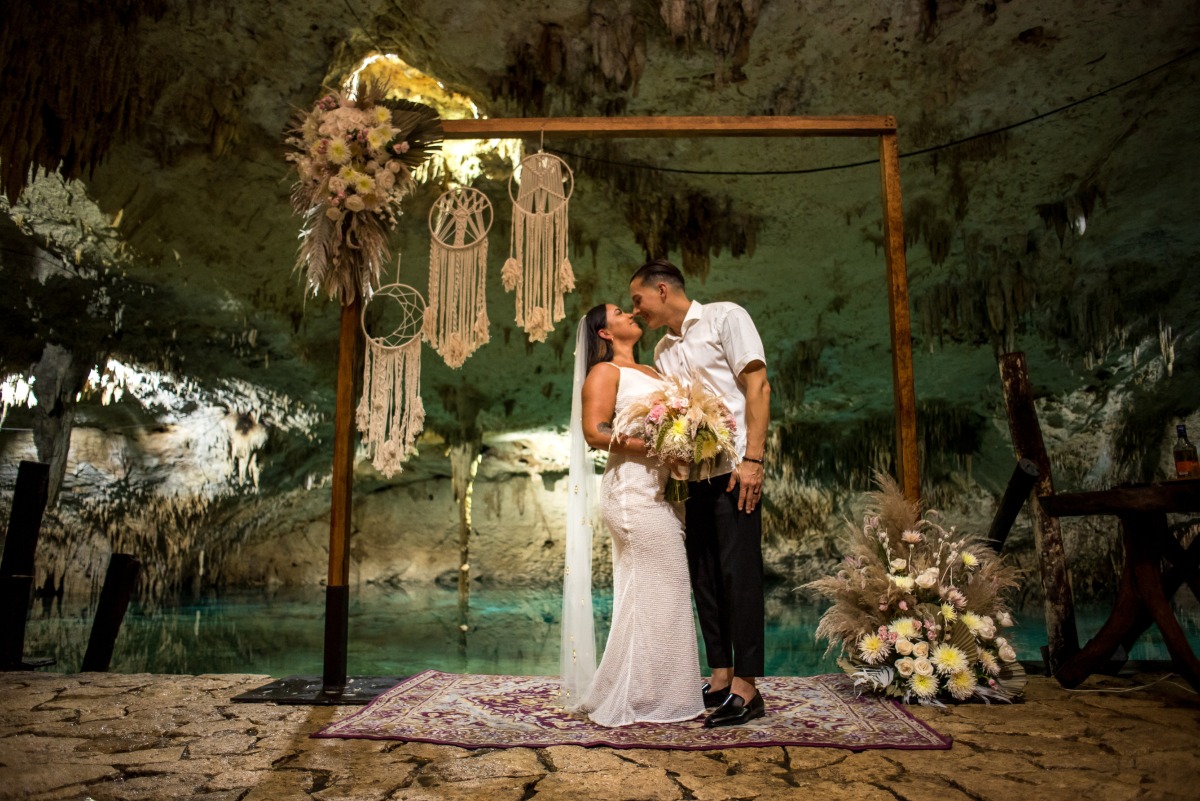This color photograph captures an intimate moment of a wedding ceremony set in an enchanting cave system, illuminated by artificial lighting. The couple, who appear to be Hispanic, stands closely together on a stone platform covered by a Persian rug, framed by an elaborate wooden archway. The bride, in a floor-length sleeveless wedding dress, and the groom, in a white button-up shirt with black slacks, black loafers, and no socks, are almost kissing, with the groom's arm gently around the bride's midsection. Above them, stalactites hang from the cave roof, and a shimmering blue pool of water lies behind them. The archway is adorned with large floral arrangements and intricate Native American dreamcatchers, including one in the shape of a crescent moon and another with a tree motif, crafted from macramé. The earthy tones of the cave and the aqua hues of the water create a magical, romantic atmosphere.